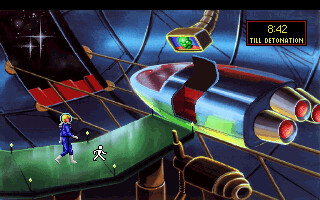The image is a detailed pixel art screenshot from a video game set in a space environment. At the center, a bullet-shaped spaceship with an open top door reveals its blue and silver interior. The ship's design includes three rockets positioned at the back, colored gray with red accents. A green pathway extends to the left from the ship, where a character in a blue spacesuit with white boots and gloves, and a bubble helmet showcasing blonde hair, is walking towards the ship. Above the spaceship, a television screen displays an alien figure, possibly conveying a message. A black rectangle with a red border at the upper right corner of the image shows a countdown clock reading "8:42 till detonation" in yellow font. The background features a space scene on the left with white stars contrasted against black, while the rest of the backdrop is a gradient of blue shades.